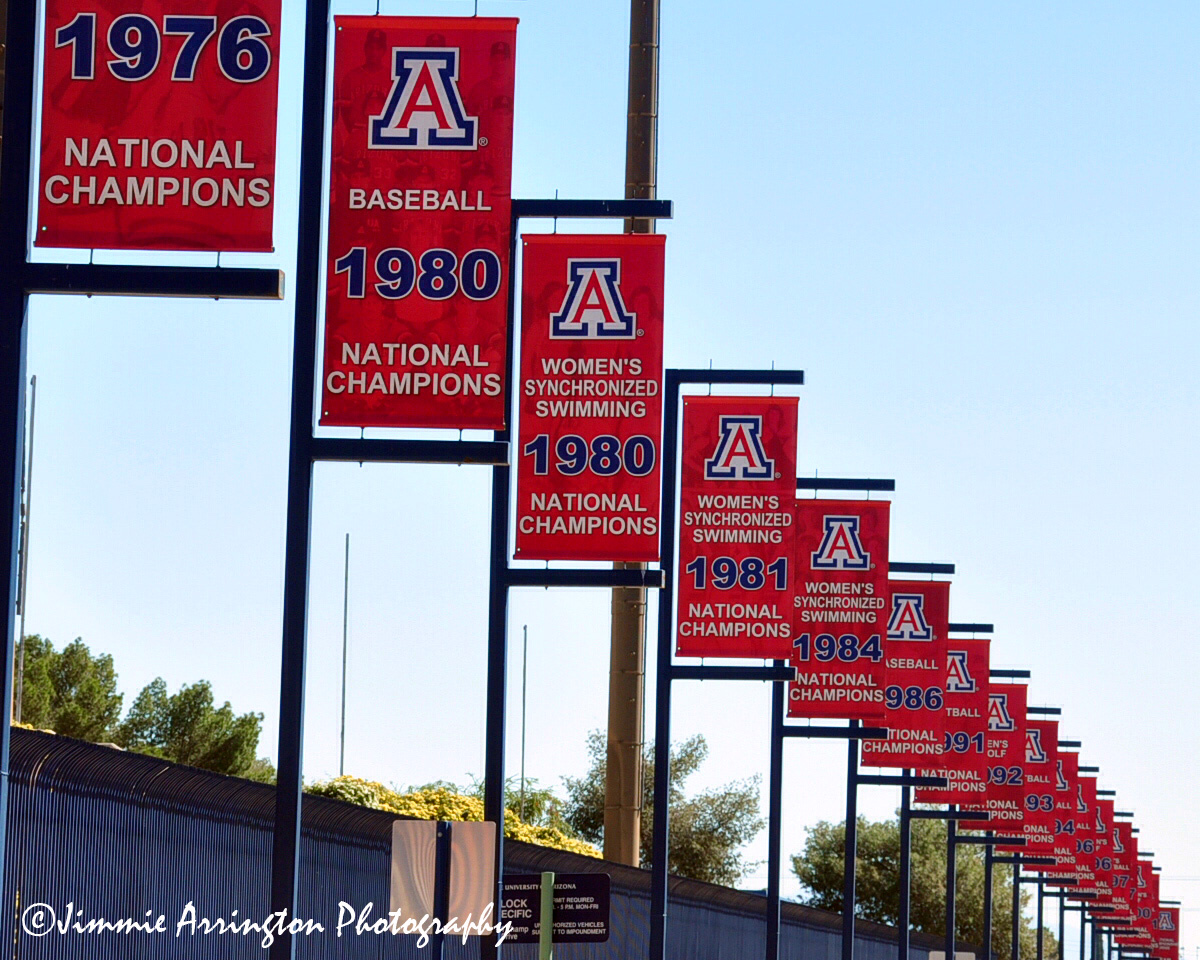In this outdoor photograph taken by Jimmy Arrington, as indicated by the white text in the bottom left corner, a clear blue sky serves as the backdrop for a row of metal poles adorned with red banners. Each pole, spaced approximately six feet apart, stretches diagonally from the top left corner into the distance towards the bottom right. These banners, celebrating the University of Arizona's sports achievements, prominently display a large capital "A" logo at the top. Among the legible banners, they acclaim various national champions: "Baseball 1980 National Champions," "Women's Synchronized Swimming 1980 National Champions," "Women's Synchronized Swimming 1981 National Champions," "Women's Synchronized Swimming 1984 National Champions," "Baseball 1986 National Champions," and "Baseball 1991 National Champions." The overlapping banners, too numerous to fully discern, suggest an extensive history of the university's sports accolades. In the foreground, the image also reveals tree foliage, with some leaves tinged yellow amongst predominantly green hues, partially covering a wall running beneath the row of banners.